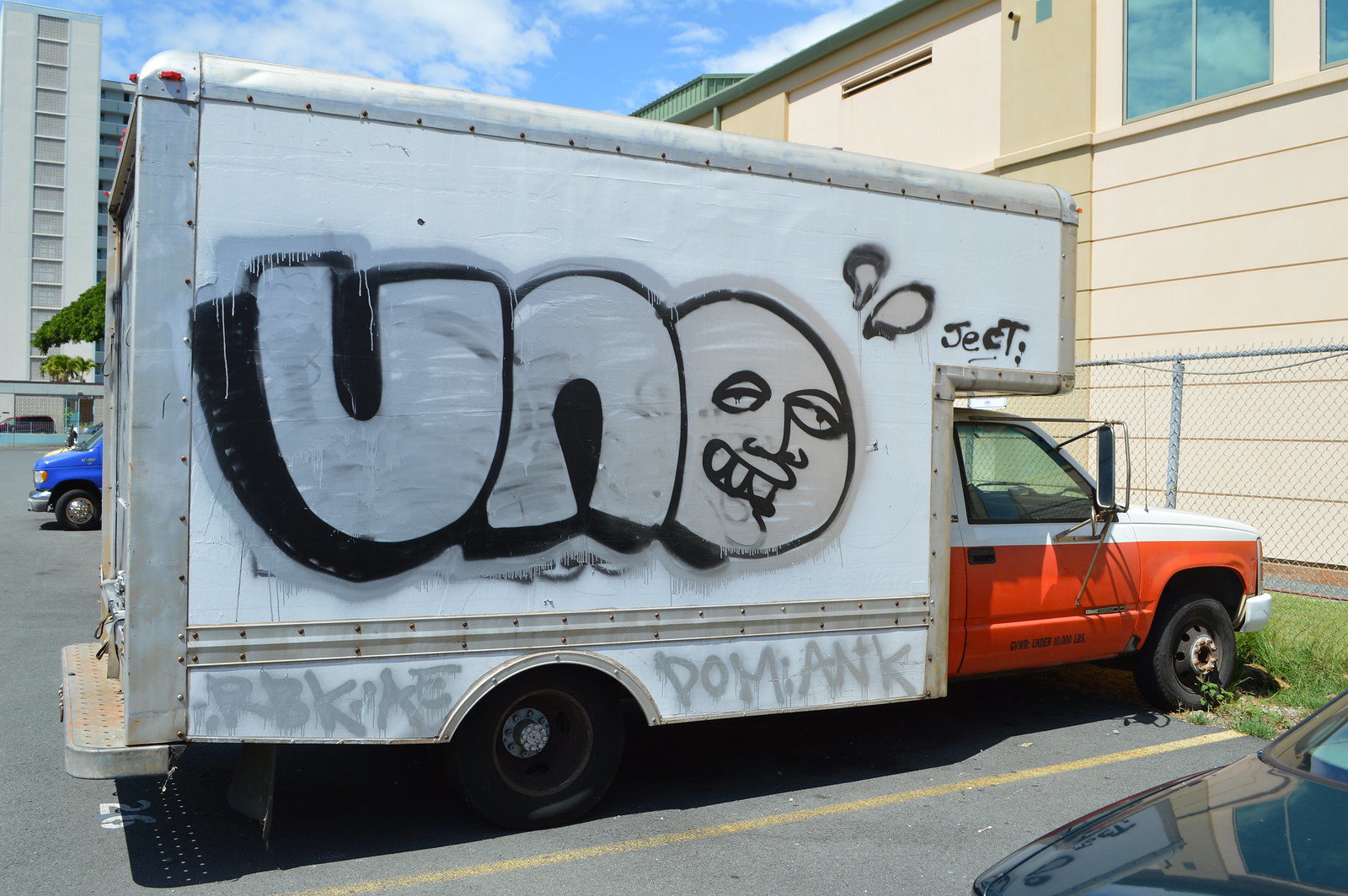This is a photograph of a large white box truck, resembling a U-Haul truck, distinguished by its orange and white color scheme. The truck’s original branding has been altered, with the back half of the box section spray-painted white and adorned with a vibrant graffiti design. The graffiti features large, bubble-lettered "UNO," where the "O" is stylized with a face exhibiting a wide, toothy grin. Below the primary graffiti, toward the wheel well, the letters "R-B-K-I-A-E" are spray-painted on one side, and "D-O-M-I-A-N-K" on the other. The scene is set in a parking lot bordered by a chain-link fence, in front of a beige house. In the background, the front of a blue truck is visible, along with tall tan buildings and a few trees. The image is captured in daylight, revealing a patch of grass and the partial view of another parked car at the right edge of the frame.